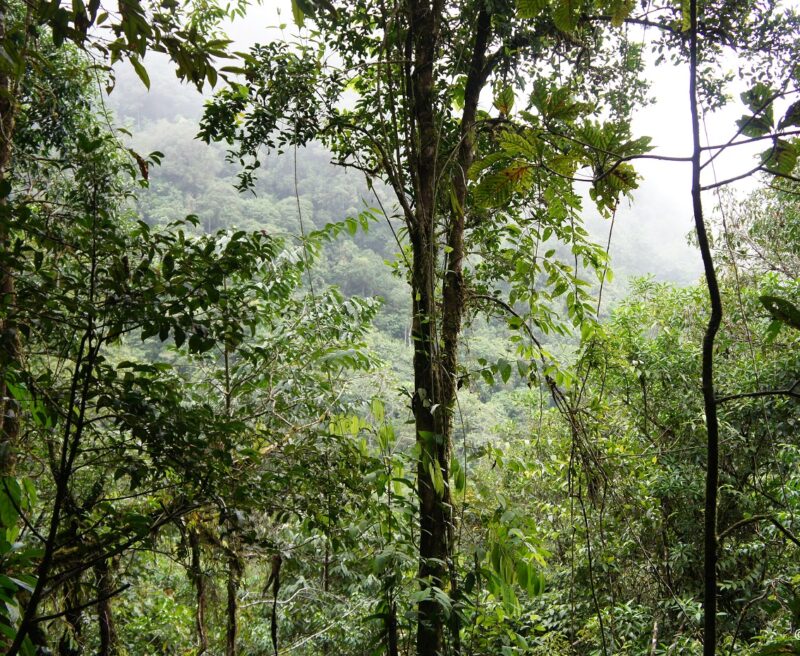This is an atmospheric photo of a densely wooded forest. The sky in the background is overcast and tinged with gray, contributing to a slightly foggy ambiance, especially concentrated on the right side of the image. The background is dominated by a tightly packed array of trees, all lush with green leaves. The landscape appears somewhat hilly or mountainous, shrouded in thick foliage, which enhances the sense of depth and seclusion within the forest.

In the foreground, the forest opens up slightly, showcasing several tall trees. One tree in the center stands out with its very narrow trunk that elegantly splits into a thin V-shape at the top, also covered in leaves. To the right of this tree, a strikingly skinny tree appears, devoid of leaves and giving the impression of a tall twig. Lower vegetation is visible, adding to the rich tapestry of greenery. The trees in the foreground exhibit sparse yet definite green foliage, hinting at a mix of deciduous and potentially tropical elements, though lacking any specific tropical indicators like palm trees. The scene is devoid of any human presence or textual elements, leaving the viewer immersed in the natural beauty and tranquil, misty atmosphere of this forest setting.